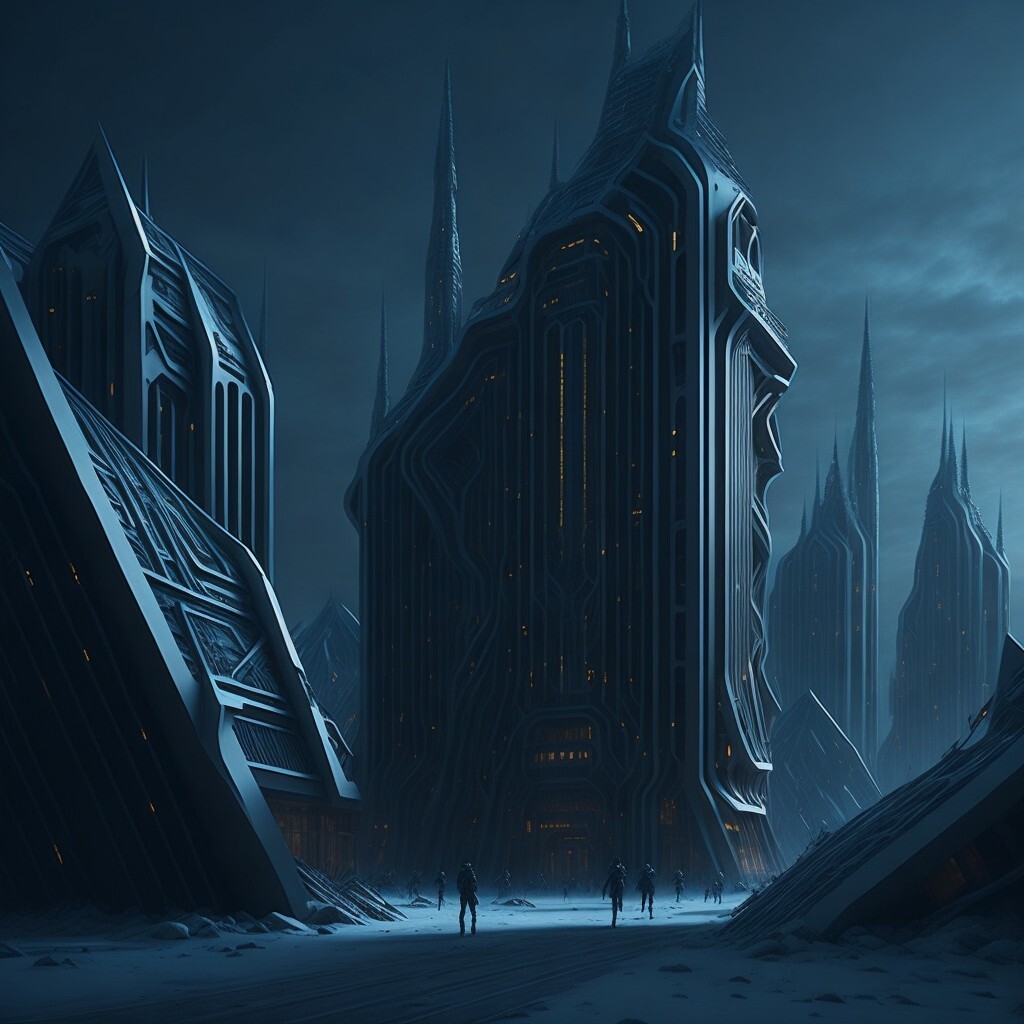The image depicts a dark, fantastical city with a strong sci-fi influence, characterized by an array of tall, black buildings with sharp, steep towers. These buildings, possibly made of an iron-like material, emit an eerie yellow light from within, casting an ominous glow through rows of windows. The night sky is equally foreboding, blanketed in dark clouds. At the base of these towering structures, numerous people appear to be in a state of panic, either walking or running along a snow-covered street. To the side of the image, a black spaceship seems to be falling, adding to the sense of urgency and chaos. The overall color palette of the scene is predominantly black with striking yellow highlights, reminiscent of a scene from a dystopian sci-fi movie such as "Dune" or "Maze Runner." The largest building, with its twin peaks, even evokes imagery similar to Batman's iconic helmet and mask, enhancing the dark, surreal atmosphere.